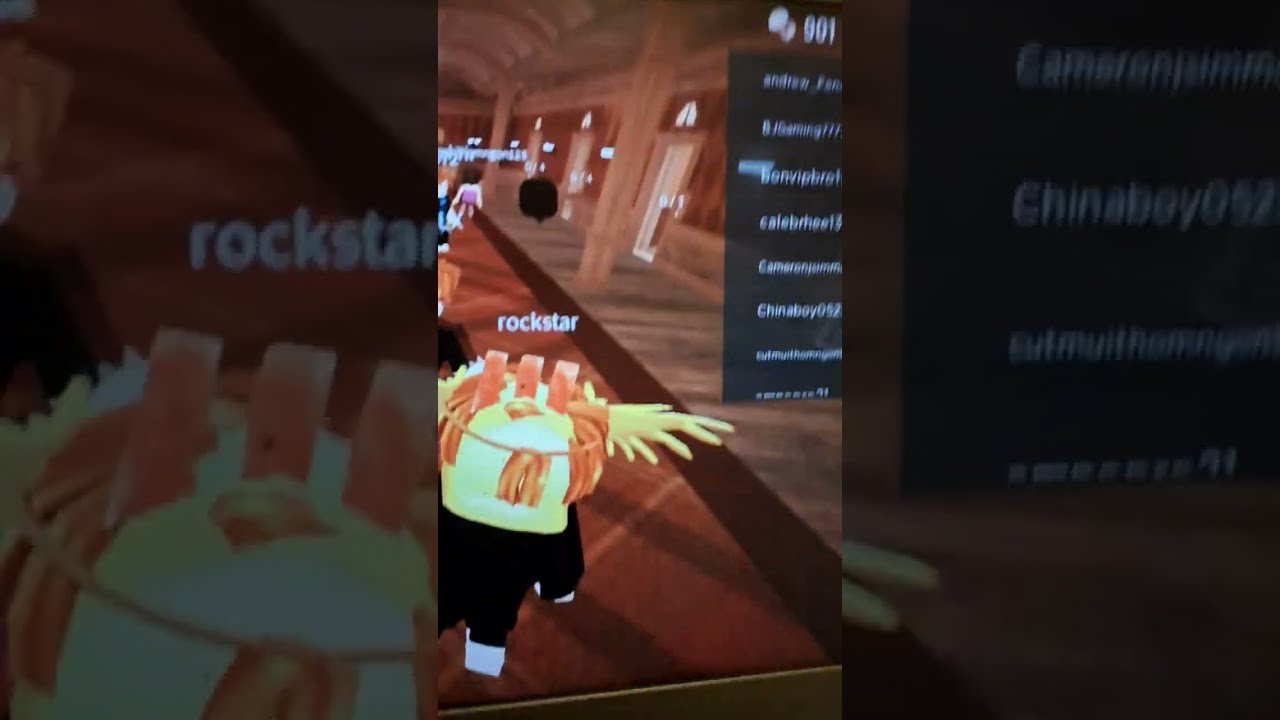The image showcases a screenshot, likely from a video game or a streaming platform on a mobile device. At the center, a long, grand hall with white pillars on the right and ornate, red, patterned carpeting stretches into the distance, evoking the grandeur of a luxurious hotel. The hall is adorned with windows dressed in curtains, with a dome-shaped ceiling above. In the foreground, a peculiar, yellowish figure with orange appendages, possibly a robot or a stylized character, stands on black legs. This character is labeled "Rockstar" in white lettering above its head. Surrounding the central image, the left and right edges darken and fragment, creating a triptych effect. The left side also features a character with stringy blonde hair, clad in black attire and white shoes, resembling a Lego figure. At the top right, a '901' label presumably signifies the number of viewers or players online, contextualized by a list of usernames denoting active participants. The overall presentation implies an interactive digital experience, captured in the portrait aspect ratio of a smartphone screen.